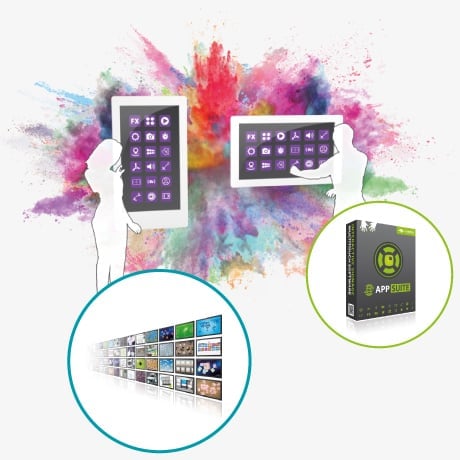A vibrant digital advertisement displays an explosion of colored powder in the background, featuring vivid shades of magenta, purple, red, gold, green, and blue. In the foreground, two tablets command attention; one positioned horizontally, and the other vertically. Each tablet boasts a sleek white border and a black screen adorned with purple and white icons. The vertically-oriented tablet showcases a white, outlined female figure, while the horizontally-positioned tablet features a similarly styled male figure. Dominating the foreground is a distinctive gray, white, and green box labeled "App Suite," encircled by a green ring. Adjacent to the green circle, a teal ring enhances the dynamic layout. Topping off the composition are several television screens displaying diverse imagery, including green grass and variously hued backgrounds, further enriching the colorful and tech-centric theme of the advertisement.